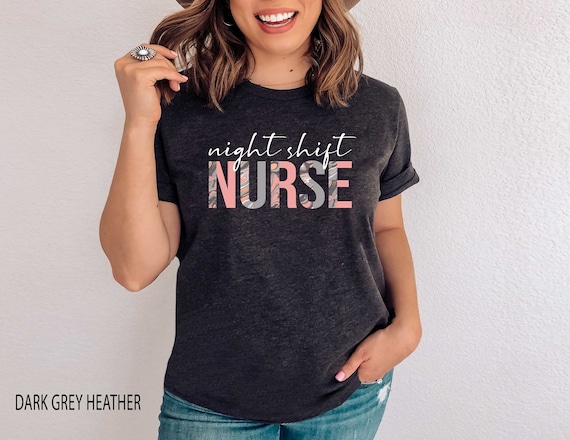In this clothing advertisement, a woman with shoulder-length brown hair and a beautiful smile is featured standing against a plain white backdrop. The image is cropped from her nose down to her waist, with her head partially cut off at the top. She is wearing a dark gray t-shirt that reads "Night Shift" in white cursive text across the upper chest, and below it, in bold, multicolored pink and blue camo print, the word "NURSE" is prominently displayed. Her right hand, adorned with a large ring on her middle finger and light pink nail polish, is raised to touch the bottom of her hair. She is also wearing blue jeans, with her left hand casually tucked into her pocket. In the bottom left corner of the image, the text "Dark Gray Heather" is visible, likely referring to the color of the shirt.